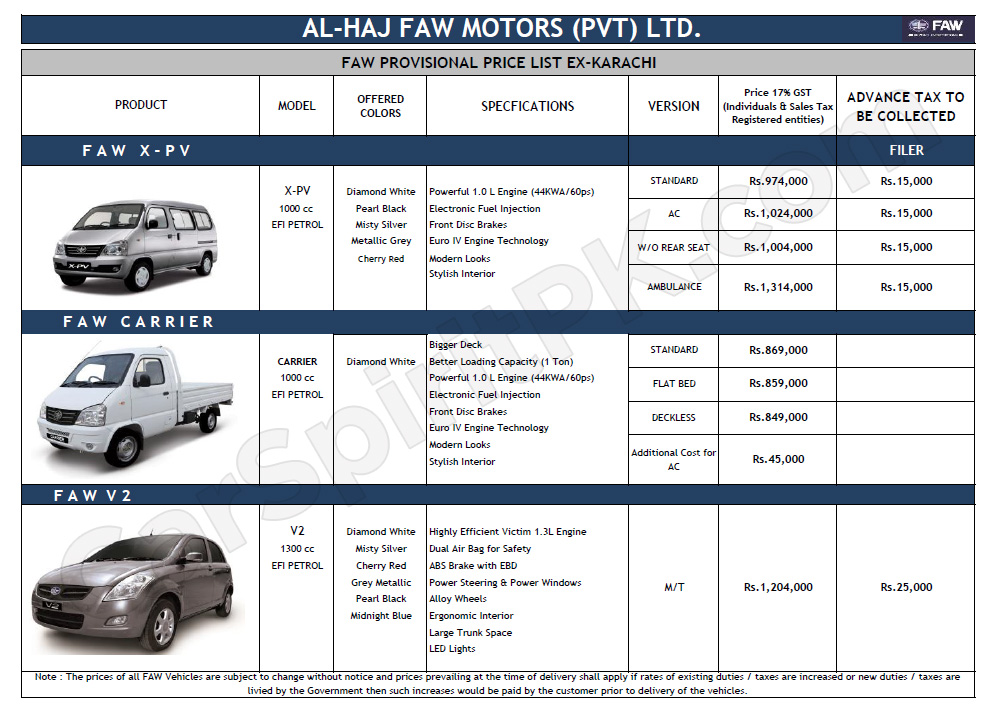In this image, we observe a detailed car listing featuring a trio of vehicles from ALHAJ FAW Motors (PVT) LTD. At the top, a prominent header reads "ALHAJ FAW Motors (PVT) LTD" followed by the title "FAW Provisional Price List - X Karachi." Below, the list showcases three distinct car models along with their specifications and available colors.

The first vehicle is the FAW XPV, specifically the XPV 1000cc EFI Petrol model. It comes in five color options: Diamond White, Pearl Black, Misty Silver, Metallic Gray, and Cherry Red. 

The second vehicle listed is the FAW Carrier, identified as the Carrier 1000cc EFI Petrol. This model is available solely in Diamond White.

The third vehicle is the FAW V2, with a more powerful 1300cc EFI Petrol engine. This model offers a broader palette of colors, including Diamond White, Misty Silver, Cherry Red, Gray Metallic, Pearl Black, and Midnight Blue.

Each vehicle description is accompanied by specifications, different versions, and respective prices. Additionally, there is a section detailing the advance tax to be collected for each model. 

At the bottom of the image, a note indicates that the prices for all FAW vehicles are subject to change without notice. It specifies that the prices prevailing at the time of delivery will apply and any increases in duties or taxes mandated by the government will be payable by the customer prior to the vehicle's delivery.

The background of the image is predominantly white, accentuated by navy blue bars that highlight each vehicle's description.